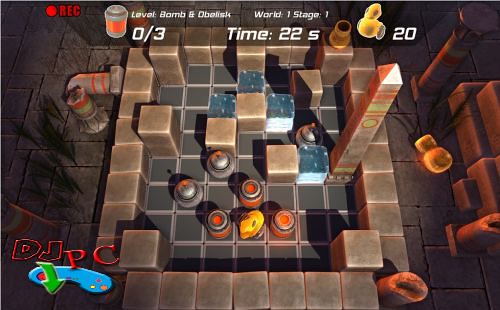The image depicts a nostalgic, top-down view of a strategy puzzle video game screen, showcasing a modern aesthetic far removed from the classic 8 or 16-bit graphics. The interface includes a stone square enclosure, scattered with various obstacles such as bombs, water blocks, and a towering obelisk—all set against a solid gray board floor that forms the maze's grid-like structure. In one corner, a rubber ducky icon with the number 20 is visible, hinting at an objective. 

The heads-up display reflects several critical pieces of information: "World 1, Stage 1" is prominently displayed, indicating the level and stage. The phrase "Level: Bomb and Obelisk" is featured in white text at the top, alongside a timer reading "22 seconds." Additionally, there's a counter displaying "0 of 3." On the lower left corner, bright text reads "DJ PC," accompanied by a PlayStation-style control interface outlined in a red font, featuring multi-colored buttons and a "REC" symbol with a red dot, which indicates recording is active. A downward green arrow is positioned beside this controller logo, further accentuating the interactive elements of gameplay. The detailed environment and UI elements illustrate a compelling blend of nostalgic design and modern strategy mechanics.